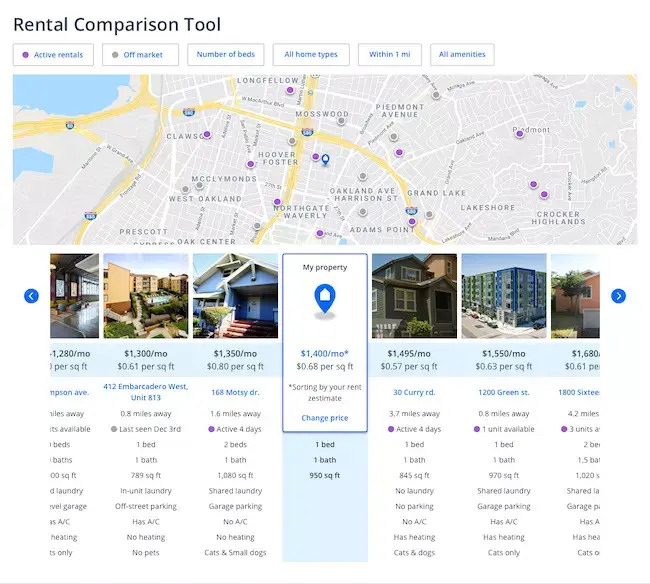The image presents a rental comparison tool on a white background with black text positioned in the top left corner, labeled "Rental Comparison Tool." Beneath the heading, there are six clickable buttons, each framed in blue with blue text inside. The buttons are labeled as follows: "Active Rentals," "Off-Market," "Number of Beds," "All Home Types," "Within 1 MI," and "All Amenities."

In the upper left section of the image, there is a Google Maps screenshot showcasing a notable blue area representing a large lake. Major roads, depicted in white, resemble interstates, while smaller white lines indicate secondary roads. Scattered across the map are gray markers pinpointing various neighborhoods with labels such as West Oakland, McKinley Woods, Grand Lake, Lakeshore, and Crocker Highlands, with the latter ironically not being near a lake.

At the bottom section of the image, there is a list of rental properties with their respective prices. The displayed prices are $1,300, $1,350, $1,400, $1,495, $1,550, and $1,680. Remarkable commentary is made on the high rental cost of a one-bedroom, one-bathroom unit listed at $1,400, with exclamations comparing the prices to more affordable mortgage rates in other regions such as Michigan. The comment highlights the lack of amenities, as some rentals are noted to have no air conditioning or heating.